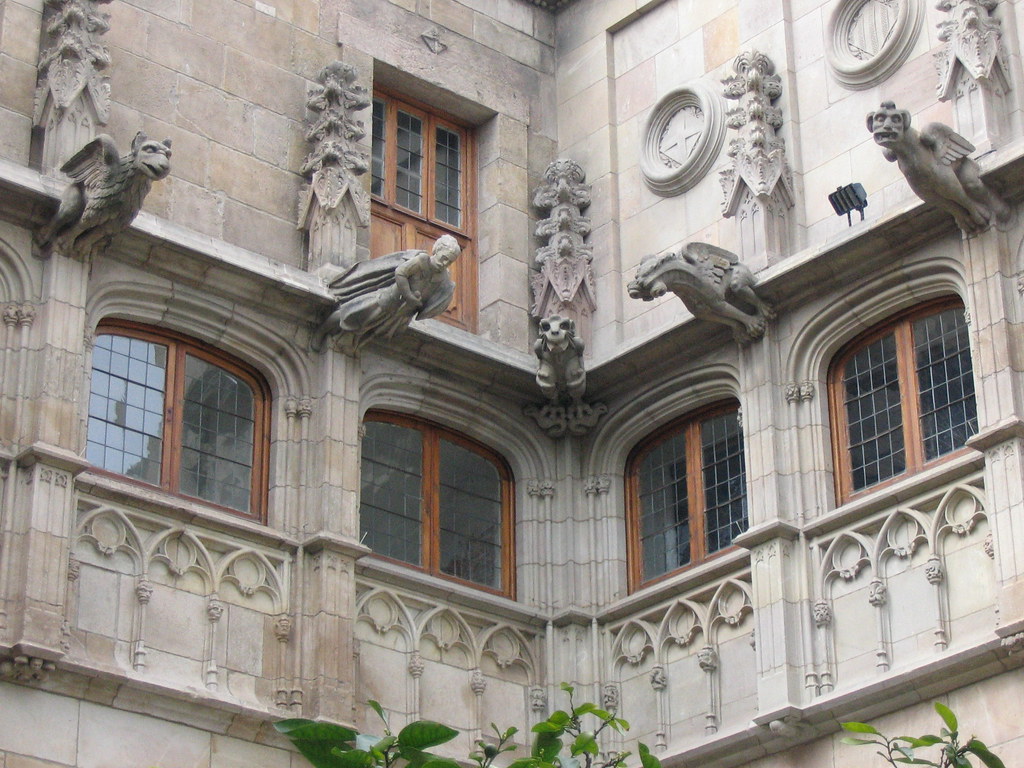The image depicts a section of an ornate, multi-story building, characterized by its Gothic or Neo-Gothic architectural style. The edifice, composed predominantly of concrete and stone with a gray-brown hue, features intricately carved stone details and statues that adorn its surface. On the first floor, there is a series of large, wood-framed windows, each segmented into smaller square panes by black net-like lines. Above these windows are various gargoyle figures, including what appear to be an angel, a dragon, and other winged creatures. The second floor includes additional statues and a wooden door with similar window designs, flanked by smaller carved details. The door seems unusually positioned as it opens onto nothing, lacking a balcony. The building corners are visible, giving the impression of standing in a courtyard. Vegetation such as green leaves and small trees enhances the scene, contrasting with the building's solid, stony appearance.